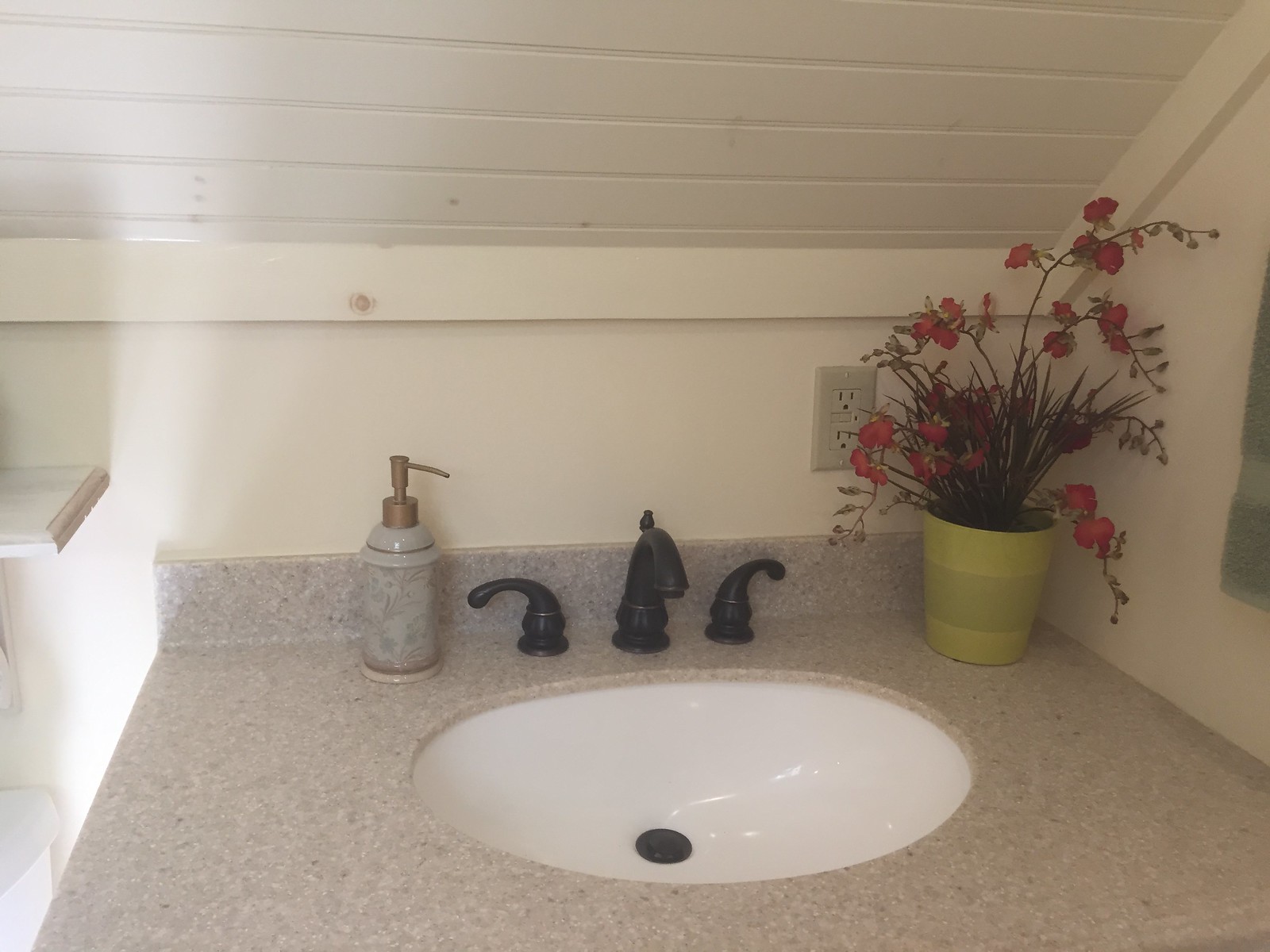The image showcases a small, cozy bathroom with an A-frame type ceiling, crafted from horizontal wooden slats and painted white. The ceiling is bordered by a thin wooden trim, also painted white. The wall below and to the right, angled upward with the ceiling, are similarly white, creating a bright and clean ambiance. 

Central to the image is a compact white sink resting on a tan granite countertop, which features flecks of black for contrast. The sink is equipped with a sleek black faucet, matching black handles, and a black drain cover, adding a modern touch to the rustic setting. 

On the left side of the sink, a white ceramic soap dispenser adorned with a gold pump, a gold line at the top, and an intricate gold motif, adds an elegant detail. In the back right corner of the sink sits a cheerful yellow metal pot containing vibrant red flowers, bringing a pop of color and life to the space.

Partially visible above the sink to the left is a shelf, and just below it, the corner of a white toilet is peeking into the frame. The entire scene exudes a blend of rustic charm and contemporary elegance, making the small bathroom feel both inviting and stylish.